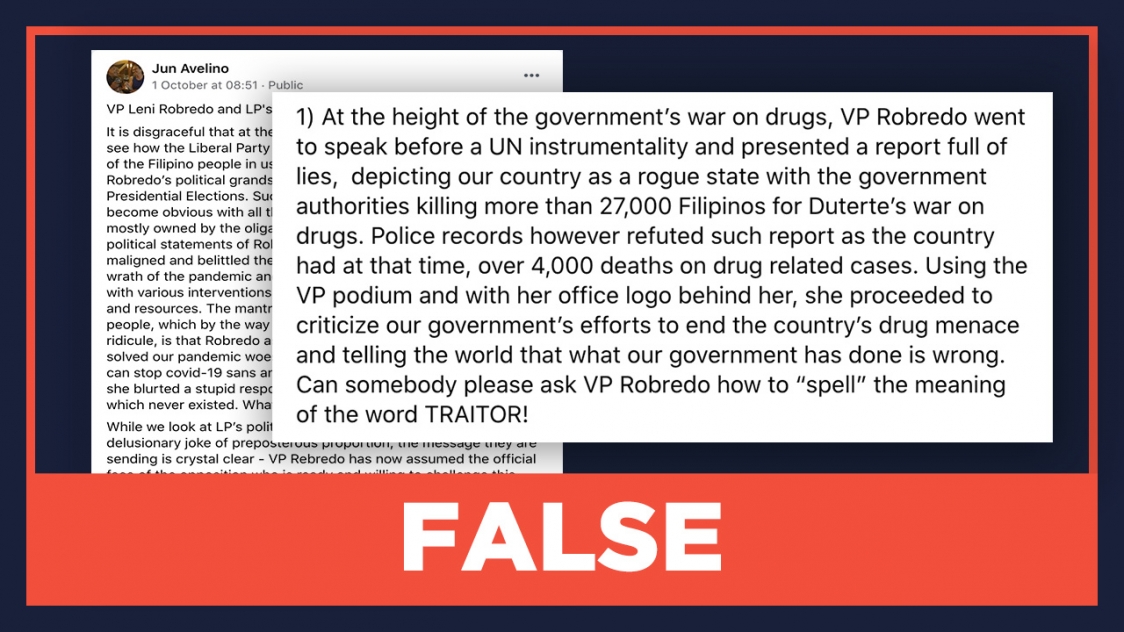The image features a background in a deep, majestic blue color, accentuated with a striking red outline. At the bottom, large white letters spell out the word "FALSE." Superimposed on the background are two screenshots of different posts containing written content. 

The primary post in the background, authored by Jun Avellino, was made on October 1st at 8:51. The specifics of the text are not entirely visible, but it’s clear enough to gather context. In the foreground, there is a smaller screenshot displaying a post whose author is not visible. This post contains a detailed critique of Vice President Robredo's actions during the height of the government's war on drugs.

The text of the smaller screenshot reads: 

"At the height of the government’s war on drugs, VP Robredo went to speak before a UN instrumentality and presented a report full of lies depicting our country as a rogue state with the government authorities killing more than 27,000 Filipinos for Duterte’s war on drugs. Police records, however, refuted such a report as the country had, at that time, over 4,000 deaths on drug-related cases. Using the VP podium and with her office logo behind her, she proceeded to criticize the government’s efforts to end the country’s drug menace and told the world that what our government has done is wrong. Can somebody please ask VP Robredo how to spell the meaning of the word TRAITOR?"

This image conveys a clear message that disputes the claims made in the critiquing post and labels them as false.